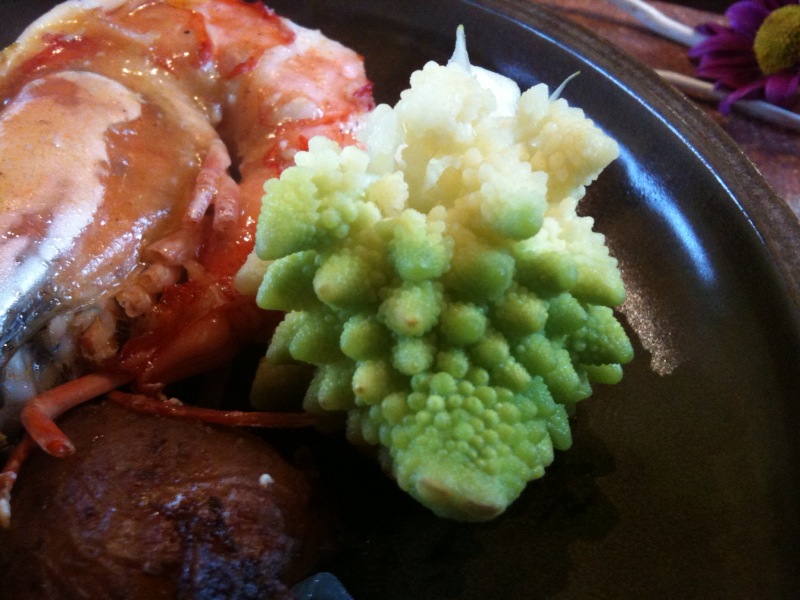This close-up photograph captures a meal presented on a large, plain black plate, set against a wooden tabletop. Dominating the left side of the plate is a sizable shrimp, its orange-red shell glistening with a layer of sauce, and its head still intact. Slightly below this is a dark brown, cooked item - possibly a potato or another root vegetable. Toward the center of the image lies a peculiar green and white vegetable, distinctively fractal in shape, somewhat resembling a hybrid between cauliflower and Romanesco broccoli. The top portion of this vegetable is mushy and soft, with white clumps merging into lime green textured bumps. In the background, a purple flower with a green center rests on the wooden table, adding a touch of color to the earthy tones. The edges of the image feature faint outlines of what might be utensils or pens, enhancing the scene with an air of casual dining.